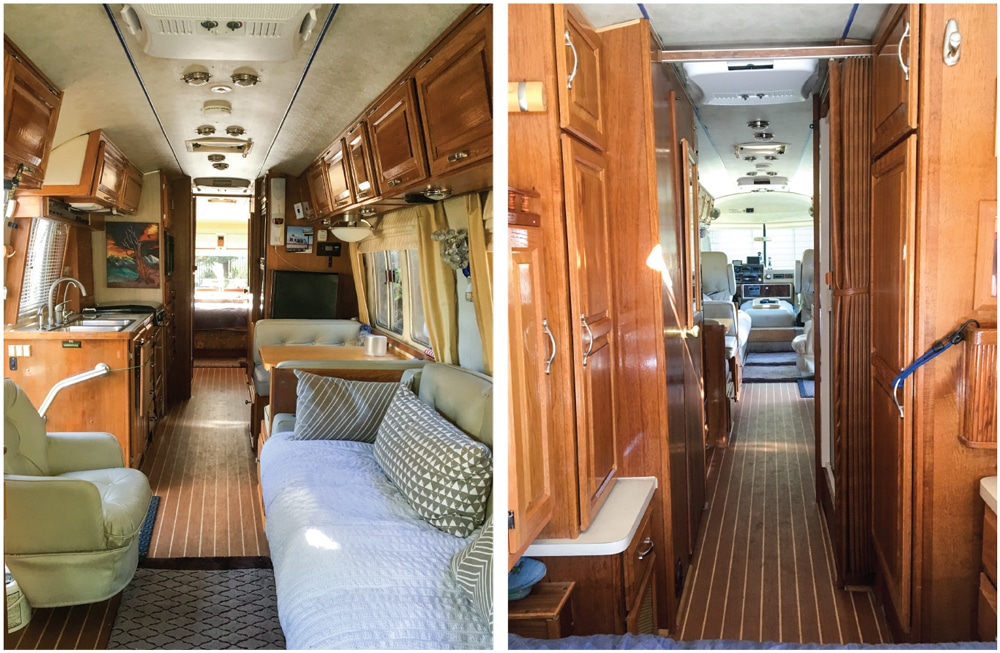This image, presented in landscape orientation, is split vertically into two panels, each showing different perspectives of the interior of a large RV, resembling a tour bus or motorhome. The left panel, facing towards the rear of the RV, showcases a cozy and well-appointed living area. Prominently featured is a gray or white leather couch on the right side, accompanied by a matching dining table with bench seats, also upholstered in a similar hue. To the left, a white swivel chair sits near the entrance door, adjacent to a kitchen sink and an oven. Above, pale cream-colored cabinets, adorned with silver handles, hang from the roof, which houses various lights and temperature control dials. The floor, a mix of brown and tan striped carpeting, extends toward the far end where bedroom windows allow daylight to stream in.

In contrast, the right panel offers a view towards the front cabin area from the rear of the RV. Here, an array of wooden cabinets lines both sides of the hallway, maintaining a cohesive warm wood aesthetic throughout the motorhome. These cabinets, equipped with simple metal handles, provide ample storage. The floor continues the theme with similar brown, striped carpeting, leading toward the driver's area. The cockpit, visible in the distance, features captain's chairs and a small table for convenience, as well as various control panels integrated into the design. The entire interior exudes a blend of comfort and functionality, making it ideal for travel.